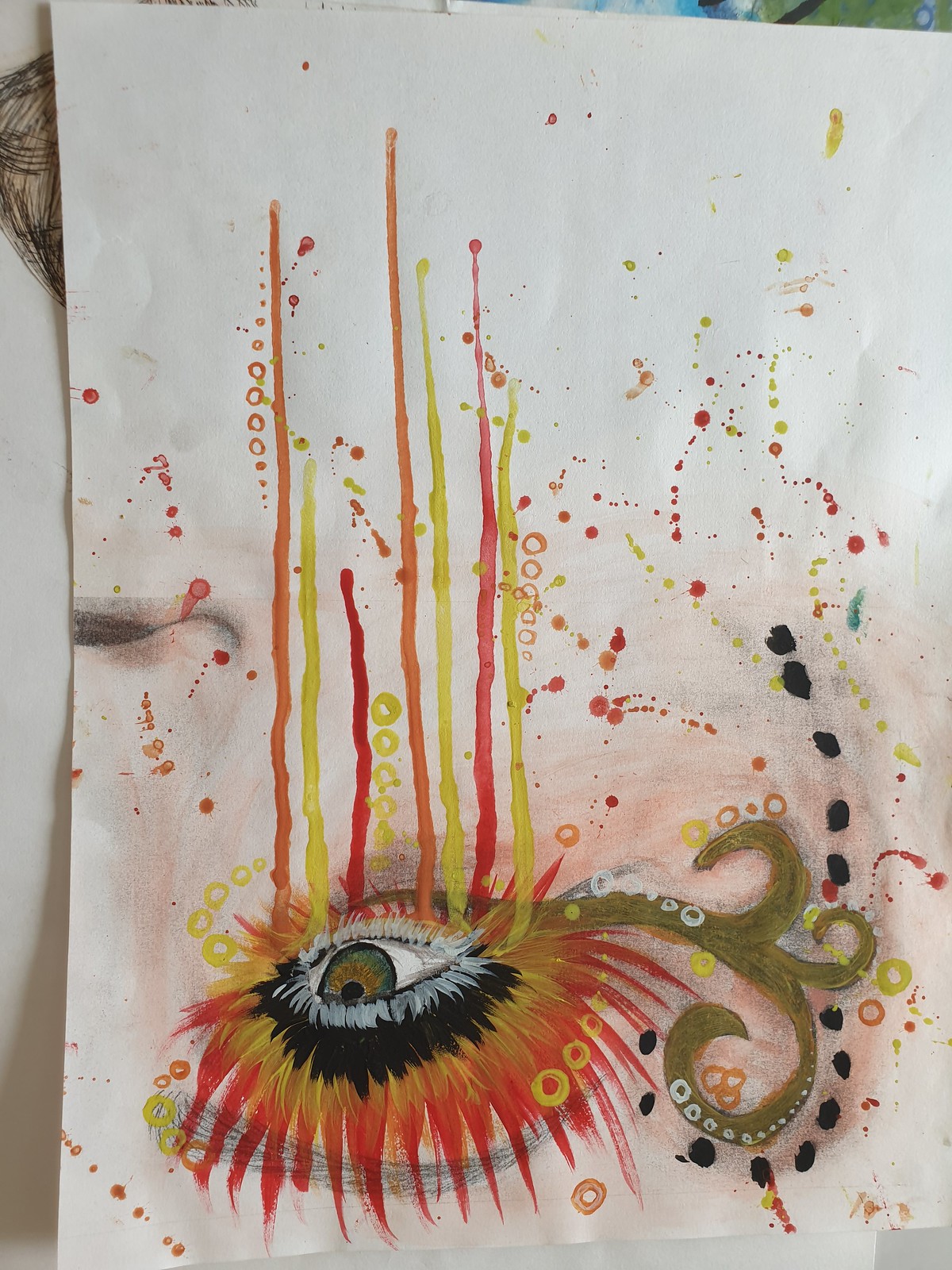A piece of white paper features a striking, surreal illustration centered around a single eye located near the bottom. The eye is artistically adorned with deep black eye shadow, creating a bold and dramatic effect. Surrounding the eye are vibrant yellow and red lashes, adding an intense and fiery contrast. Emerging from the right side of the eye are brown tentacle-like curves, enhancing the otherworldly feel of the artwork.

In a defiance of gravity, a cascade of colors appears to drip upwards from the eye. On the left, the hues transition from a muted orange to yellow, to a vivid red, and repeatedly cycle through these colors as they ascend. On the very far right side of the paper, clusters of black dots add texture to the composition.

Scattered across the paper are large spiders rendered in a spectrum of colors, contributing to the overall surreal and slightly macabre atmosphere.